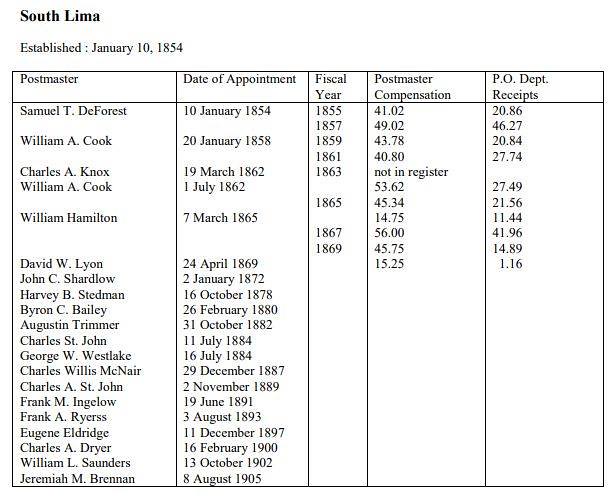The image displays a detailed black and white chart titled "South Lima, established January 10, 1854" in the upper left corner. The chart, set against a simple white background, features black text and black lines forming borders to organize the information. Five columns span across the chart. The first column lists the names of various postmasters, beginning with Samuel D. T. De Forest on January 10, 1854, with his fiscal year 1855 pay listed as $41.02 and receipts at $20.86. This system continues with other postmasters, such as William Cook who was appointed in January 1858, receiving $43.78 in compensation and bringing in $20.84 in receipts. Each subsequent row provides similar details for a full dozen postmasters, including their dates of appointment, fiscal years, compensation figures, and post office department receipts, extending through to the last recorded date of August 8, 1905.